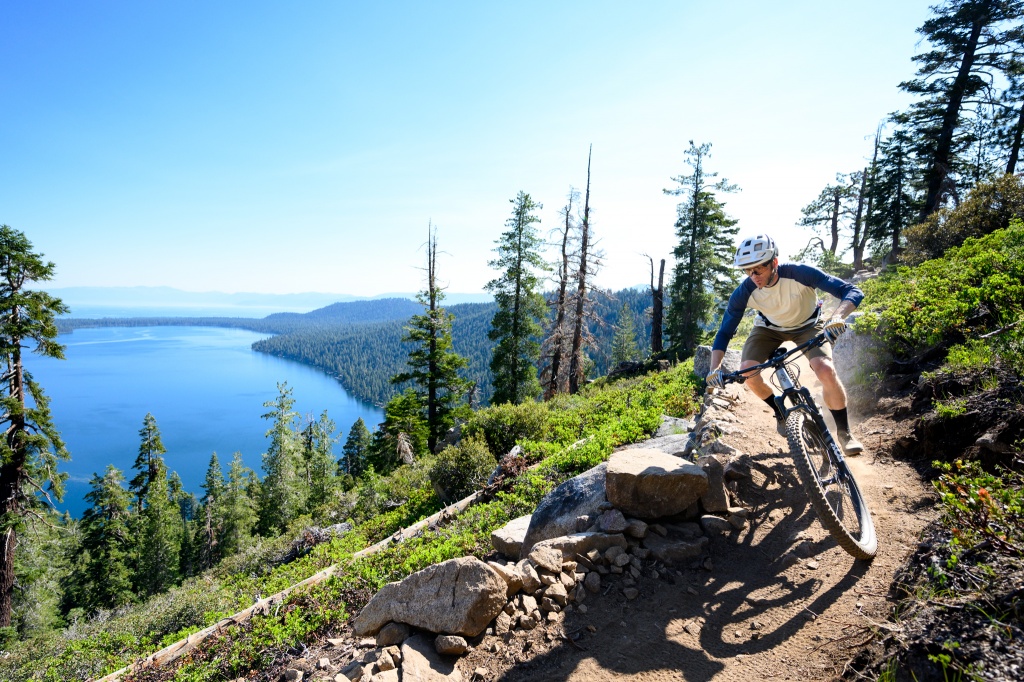This horizontal photograph beautifully captures a scenic mountain biking adventure. On the right side of the image, a man in a blue-sleeved, white-torso long-sleeve shirt and bike shorts is riding a black mountain bike with chunky tires down a narrow, dirt trail. The trail, about three to four feet wide, switchbacks down the hillside and is flanked by rocks and green vegetation, which includes trees and lush undergrowth. To the left, the rugged terrain sharply contrasts with the serene, deep blue lake in the background. The lake's waterway lies far below, accentuating the steepness of the descent. In the distance, a lush forest filled with numerous trees covers the hillside, adding to the pristine beauty of the landscape. The sky features a gradient transitioning from blue in the top left corner to a lighter hue near the bottom right, behind the cyclist. The detailed and picturesque scenery, reminiscent of places like Oregon, makes this image a vivid depiction of an exhilarating mountain biking experience through nature’s splendor.